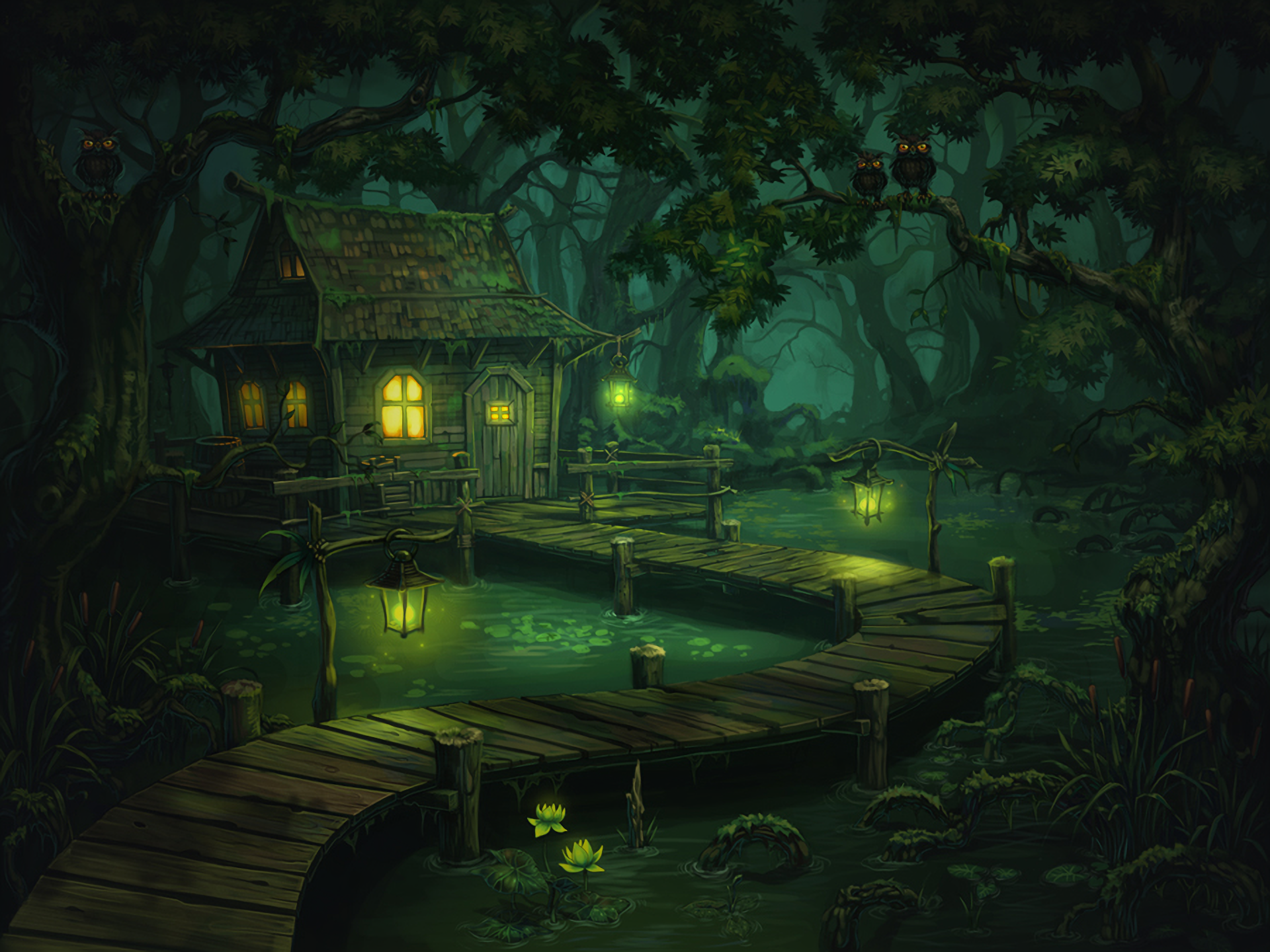This computer-animated image depicts a dark, atmospheric scene reminiscent of a mysterious bayou or forest setting. Dominated by shades of black and green with sparse accents of yellow light, it evokes a nighttime ambience. Dark, leafy trees surround the scene on the left, right, and top, their branches home to three owls—two in the upper right and one in the upper left—each with piercing gold eyes. At the heart of the image is a simple wooden cabin with multiple glowing yellow windows and a small yellow window in the door, illuminating the surrounding space. A lantern hangs from the corner of the cabin, casting light onto a curved wooden boardwalk that navigates through the water below, leading from the lower left to the middle of the scene. Lanterns along the boardwalk add to the light, highlighting a few yellow flowers or water lilies near the bottom of the image. The water is calm and dotted with lily pads, perfectly complementing the dim and eerie atmosphere.